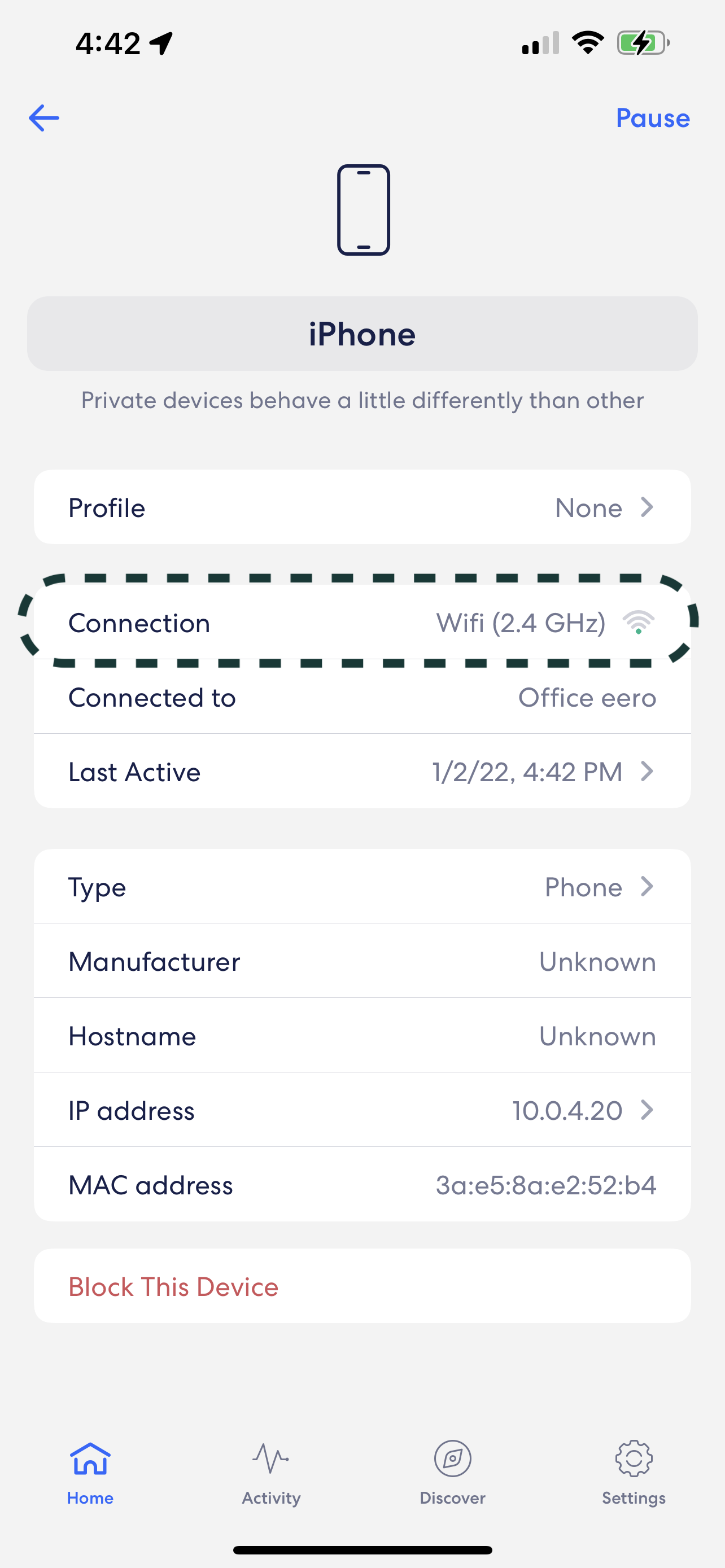The screenshot captured on an iPhone depicts a section within the device's settings, presumably under "About Phone." The background is a light shade, creating a clear contrast with the elements on the screen. At the top, a faint blue arrow indicates a navigation option, yet no specific section title is visible. Prominently displayed on the right is the word "PAUSE" in blue text, indicating a user interface element. 

Below "PAUSE," a simplistic illustration of the iPhone's shape is evident, followed by a gray bar showcasing the word "iPhone." An intriguing snippet of text states, "Private devices behave a little differently than other," which appears to be a grammatically awkward phrase. Subsequently, the detailed information regarding the phone is listed. It begins with "Profile: None," followed by "Connection: Wi-Fi 2.4 GHz," which shows a weak connection strength. This specific connection detail is highlighted with a dotted-line circle, drawing attention to the Wi-Fi status.